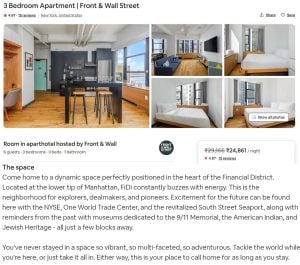This desktop screenshot appears to be a blurred image of an online listing for a rental property. The visible text at the top left in black print indicates that it is a listing for a "Three Bedroom Apartment" located at "Front and Wall Street" in Manhattan, New York. Below this, a rating of 4.31 can be discerned, though the rest of the details are not clearly legible. The interface seems to have icons that suggest options for saving or sharing the listing.
 
The image contains five pictures showcasing different aspects of the apartment. The largest image on the left appears to capture an open-plan space that combines a kitchen, dining area, a potential office nook, and access to a balcony. The remaining pictures show various areas of the apartment including the living room and the three bedrooms.

Despite the blurriness, it's indicated that the nightly rental price is 24,561 Euros. Below the images, there seems to be a description of the property reading: "Come home to dynamic space, perfectly positioned in the heart of the financial district. Located at the lower tip of Manhattan, FIDI constantly buzzes with energy. This is the neighborhood for explorers, deal makers, and pioneers. Excitement for the future can be found here with the NYSE, One World Trade Center, and the revitalized South Street Seaport, along with reminders from the past with museums dedicated to the 9-11 Memorial, the American Indian, and Jewish heritage, all just a few blocks away. You've never stayed in a space so vibrant, so multifaceted, so adventurous. Tackle the world well..."

This listing presents a uniquely vibrant and adventurous living experience in the energetic and historic Financial District of Manhattan.